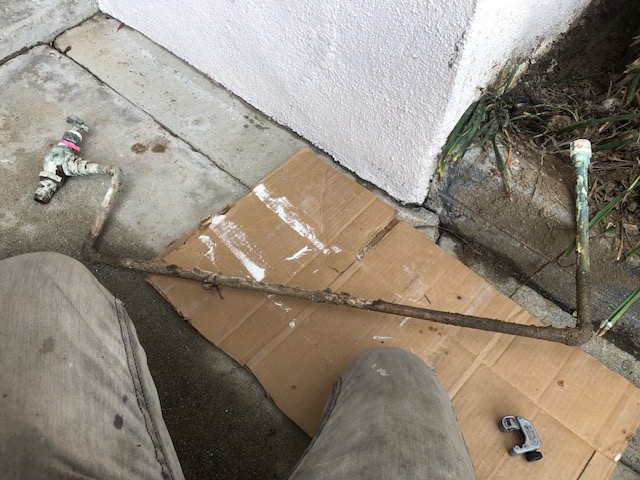In this image, a person is kneeling on a piece of cardboard placed on a light gray, cracked concrete surface. The individual is wearing a black or gray stonewashed hoodie and jeans. Their right knee rests on the cardboard, indicating they might be involved in some kind of manual work. In front of them is a long, thin metal piece with nozzles on both ends, which could be a tool used for painting.

The scene is set in front of a freshly painted, bright white stone wall. The cardboard beneath the person has traces of white paint, hinting that they might be in the process of painting or finishing up the task. Just below their left leg, the concrete appears darker, likely due to condensation from recent rainfall. Adjacent to the painted wall is a small flower bed containing dark brown and green, seemingly dead grass, adding a contrast to the otherwise clean and bright setting.

The photo is captured outside during the day, probably later in the afternoon, given the subdued lighting and minimal shadows. The overall atmosphere suggests a casual yet focused moment of work or creativity.